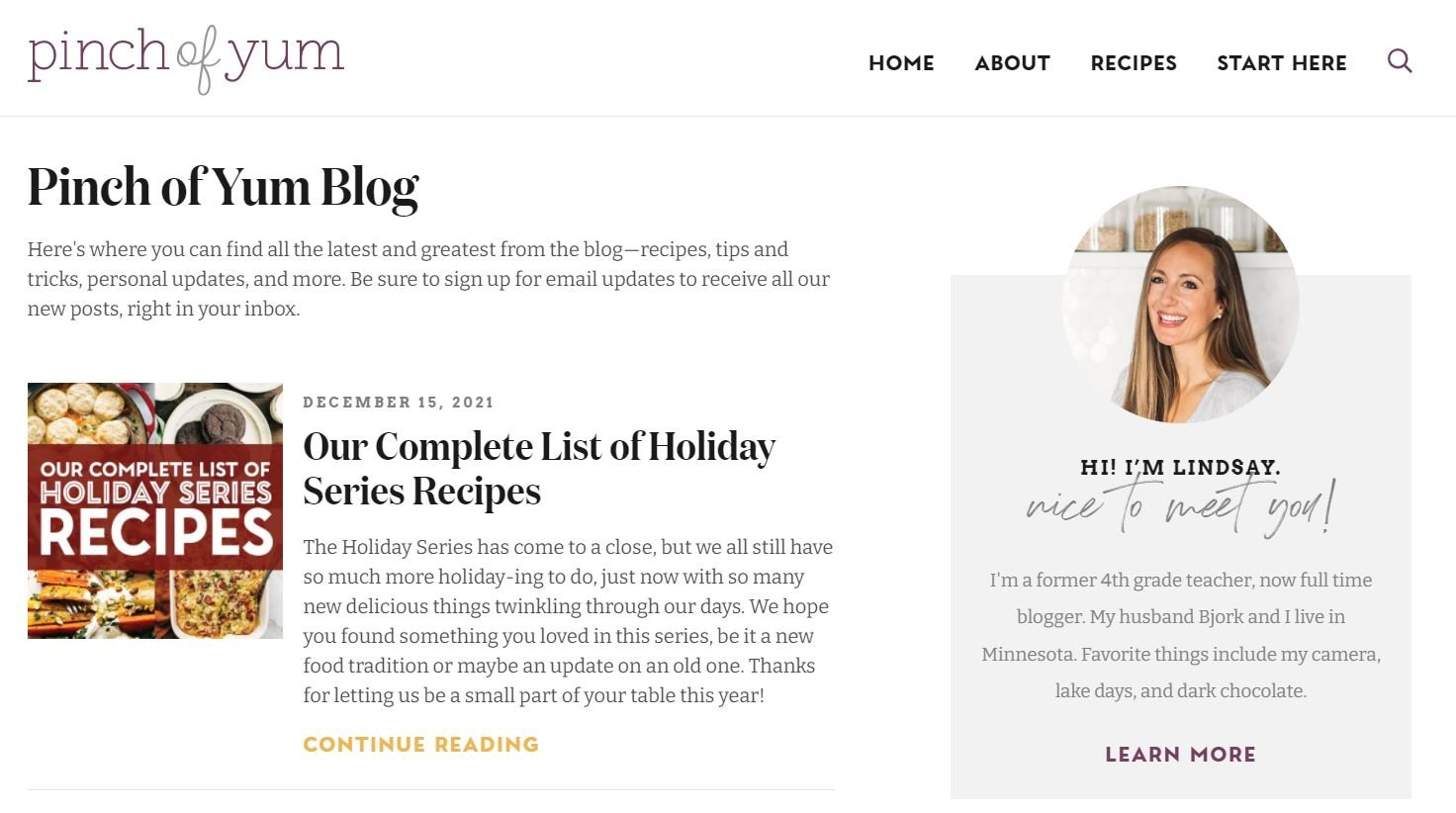In this image, we see a screenshot of a website. In the upper left corner, light gray text reads "Pinch of Yum." The upper right corner features a menu with options in bold, small gray text: "Home," "About," "Recipes," and "Start Here." A thin horizontal gray line separates the menu from the main content. Below this line, on the left side, there is very large, bold black text reading "Pinch of Yum Blog." Underneath this heading, the following description appears: "Here's where you can find all the latest and greatest from the blog: recipes, tips and tricks, personal updates, and more. Be sure to sign up for email updates to receive all our new posts right in your inbox."

On the right side of the screenshot is a photo of an attractive woman with long brown hair and fair skin. Beneath her image, in a light gray box, it reads, "Hi, I'm Lindsay. Nice to meet you."